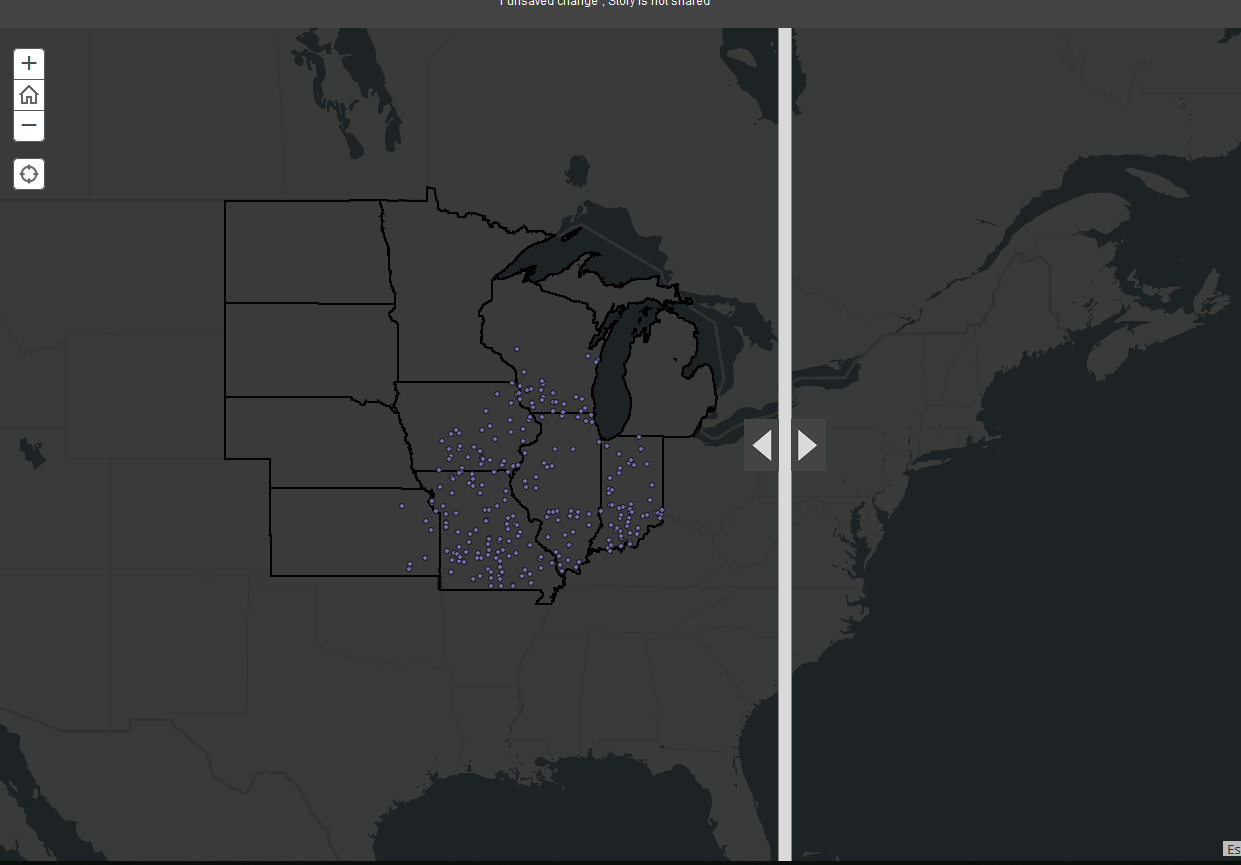This image depicts a detailed map of the United States, predominantly shaded in gray, with bodies of water appearing in a darker hue. In the top left corner of the map interface, there are several icons including a plus sign likely for zooming in, a home button depicted with a house icon, and a minus sign for zooming out. A distinct white line runs horizontally near the center of the map, accompanied by two arrows pointing left and right, respectively. Highlighted within the map are several states, outlined with black boxes, including Michigan, Wisconsin, Minnesota, Illinois, and Indiana, extending slightly beyond these regions. Numerous purple dots are scattered across these highlighted states, forming clusters that suggest the locations of specific points of interest—possibly indicating the density of a certain business or service in the Midwestern region of the United States. The detailed focus and clustering patterns highlight the significant concentration of these points within the Midwest.